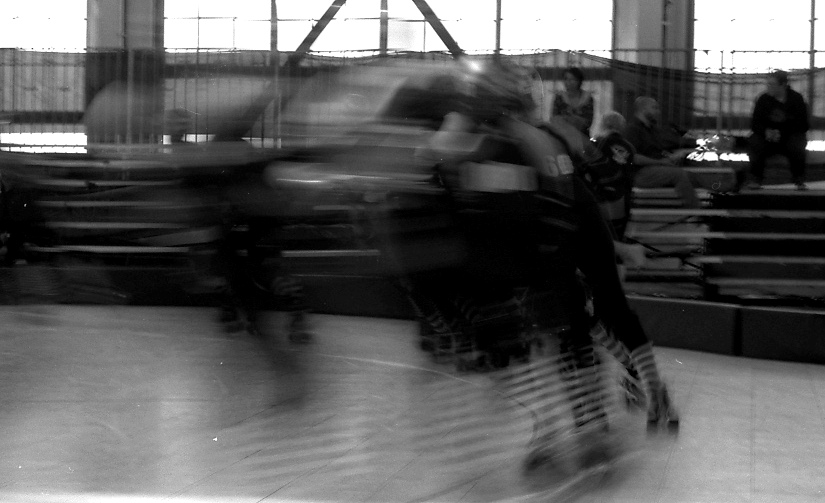The photograph is a black and white, out-of-focus image capturing the vibrant motion within an indoor roller skating rink. Dominating the foreground, a few skaters—likely two or three—wear distinctively striped socks that alternate between dark and light hues. They are equipped with quad roller skates, featuring four wheels each, and all are donned in helmets for safety. The skaters appear as blurs, their rapid movement stretching their forms into trailing streaks that flow leftward, creating an impression of swift, continuous motion. The rink itself is a rounded area delineated by clear lines, facilitating the circle-like path the skaters follow. In the background, metal railings form a boundary, while bleachers are set against the rear wall, occupied by an audience attentively watching the scene unfold. The combination of the image’s blur and lack of focus emphasizes the frenetic, dynamic environment typical of a bustling roller rink.